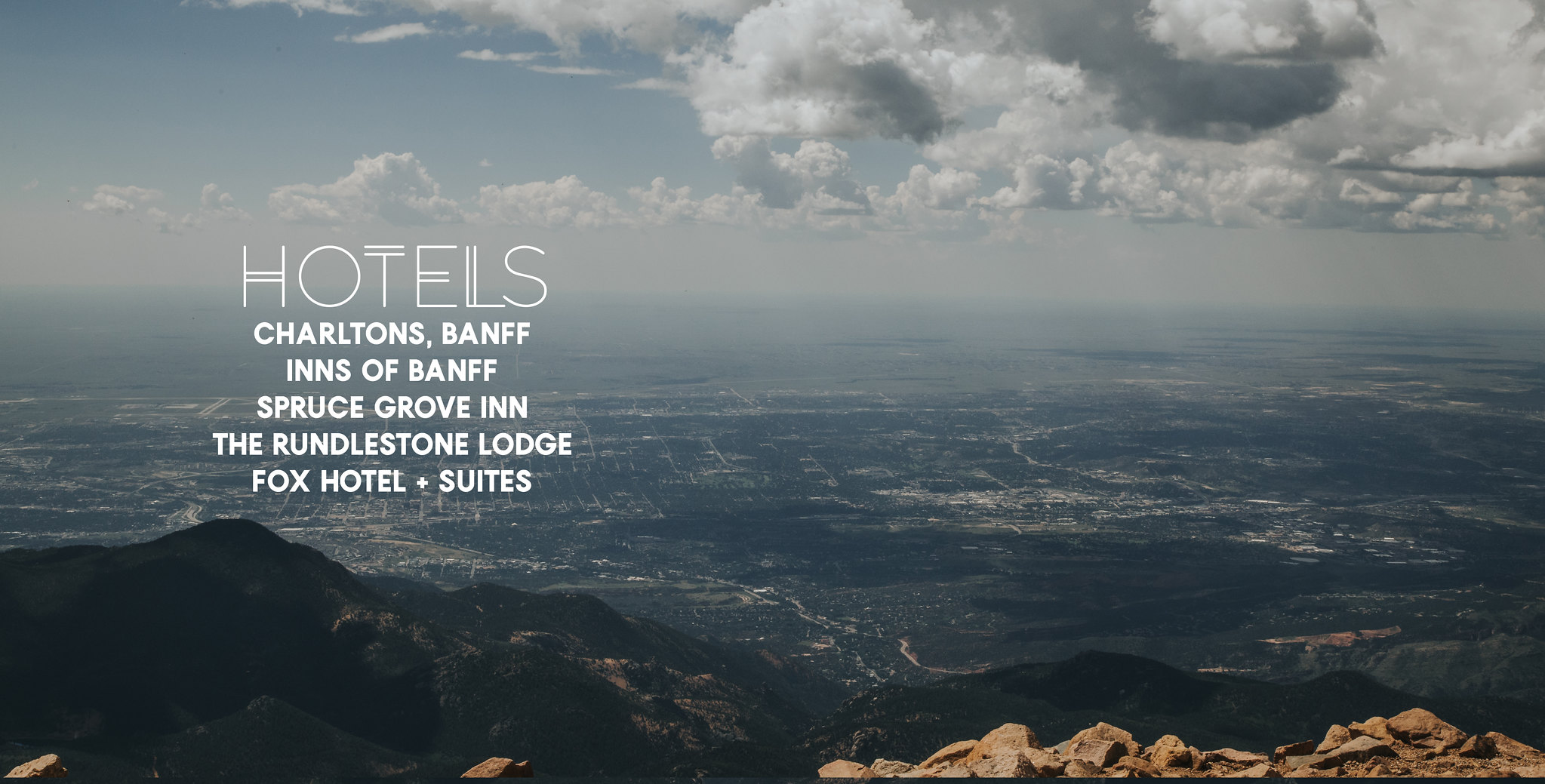This image is a high-altitude, aerial photograph capturing a scenic, mountainous landscape. The foreground features a rocky cliff with brown and tan rocks, indicative of a mountaintop terrain. Stretching out beneath this vantage point is an expansive countryside view, dotted with houses, grass, and trees, leading up to a distant, hazy horizon. The upper portion of the image showcases a light blue sky filled with clouds, particularly concentrated in the upper right area, adding to the serene and picturesque atmosphere. Overlaid on this beautiful scenery is white text listing several hotels: "Charlton's Banff Inns, Banff Spruce Grove Inn, The Rundlestone Lodge, and Fox Hotel & Suites," suggesting the image doubles as an advertisement for these accommodations despite none being visible in the photo. The overall color palette includes light blue, white, gray, black, brown, and tan, enhancing the natural beauty of the landscape.